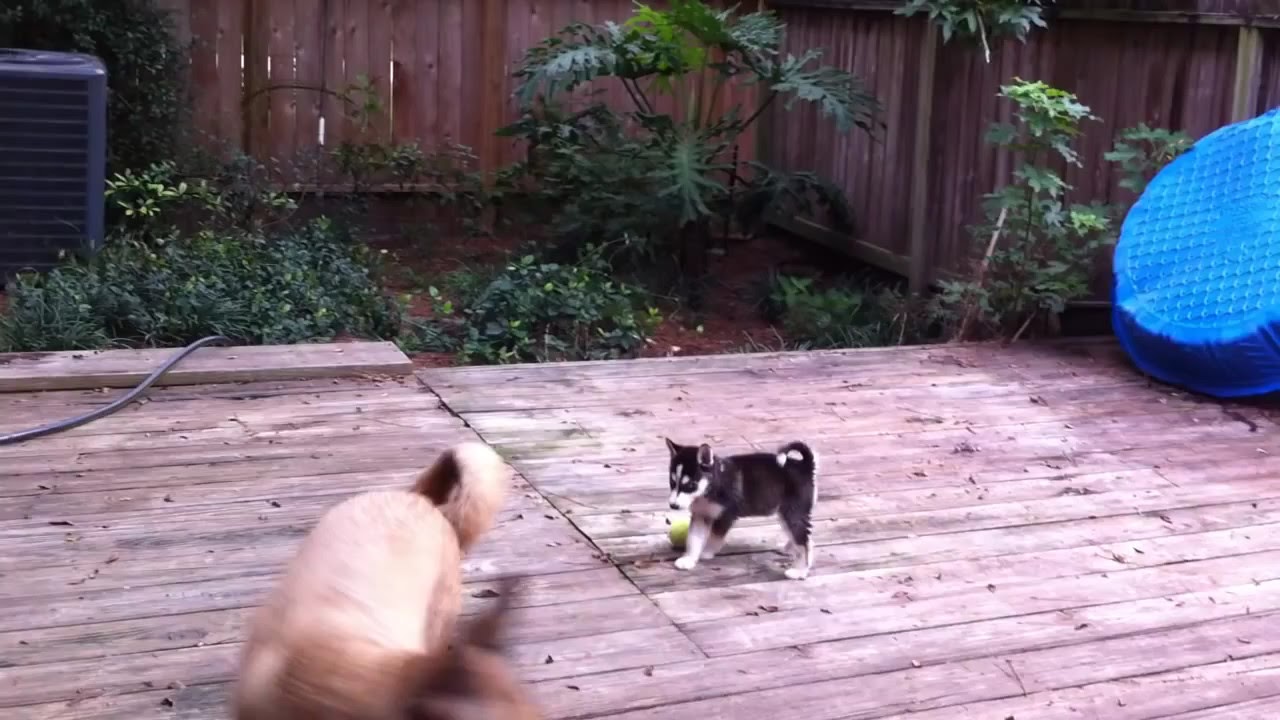In this photograph, the setting is a wooden back porch that seems to belong to someone's backyard. The deck, made of long wooden slats with a light reddish cedar hue, is scattered with leaves. The area is fenced in with light reddish cedar fencing. There are two dogs on the porch, appearing to be engaged in play. The central figure is a black and white puppy, possibly a shepherd breed, standing still and observing the other dog. This puppy has black fur on its back, head, and ears, with white fur on its muzzle and paws, and it even appears to have a small neon tennis ball nearby. The second dog is larger, brown in color, and appears blurry due to motion, suggesting it is actively moving.

In the background, there is lush vegetation, including various green bushes and tropical plants with long, fanning leaves. A blue, circular kiddie pool lies upside down on the right side of the porch, indicating it is not in use. On the top left, a large gray air conditioning unit can be seen, adding to the residential feel of the scene. A garden hose snakes its way into the vegetation, hinting at the home’s maintenance activities. Overall, the image captures a lively and homely atmosphere with playful dogs and a well-used backyard space.